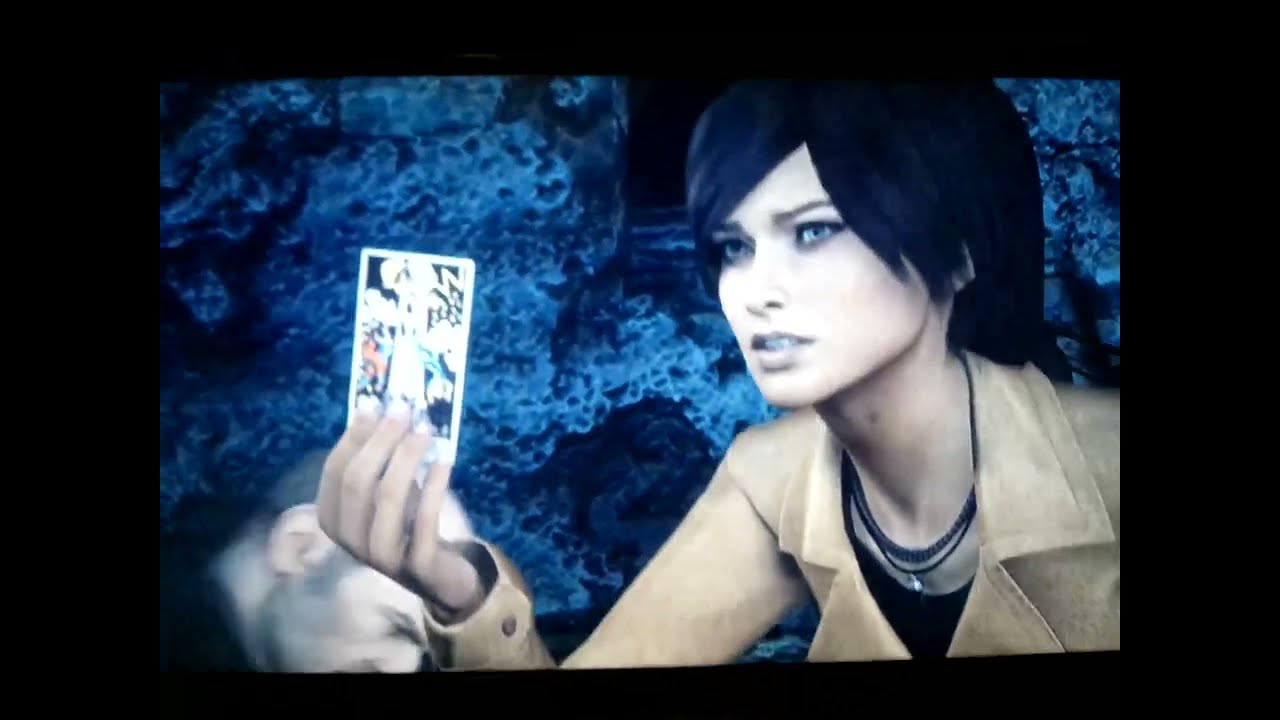This is a detailed screenshot from a video game depicting an Asian woman in her early to mid-20s with short black hair styled in a bob. She is standing and holding a card that resembles a tarot card, which she appears to be showing to someone, possibly seeking an answer. The card features a symbol or an image, likely of a tower. She is dressed in a tan leather jacket with lapels, a black shirt, and three beaded necklaces. Next to her, a white man with short grayish hair is seen sitting or kneeling down, with his head resting against what appears to be a cave wall. The background is characterized by a blue textured environment that looks like a cavern with porous, sponge-like rocks. The image captures a moment of interaction and seems to convey an atmosphere of mystery and exploration, emphasizing the detailed and immersive environment typical of a video game.